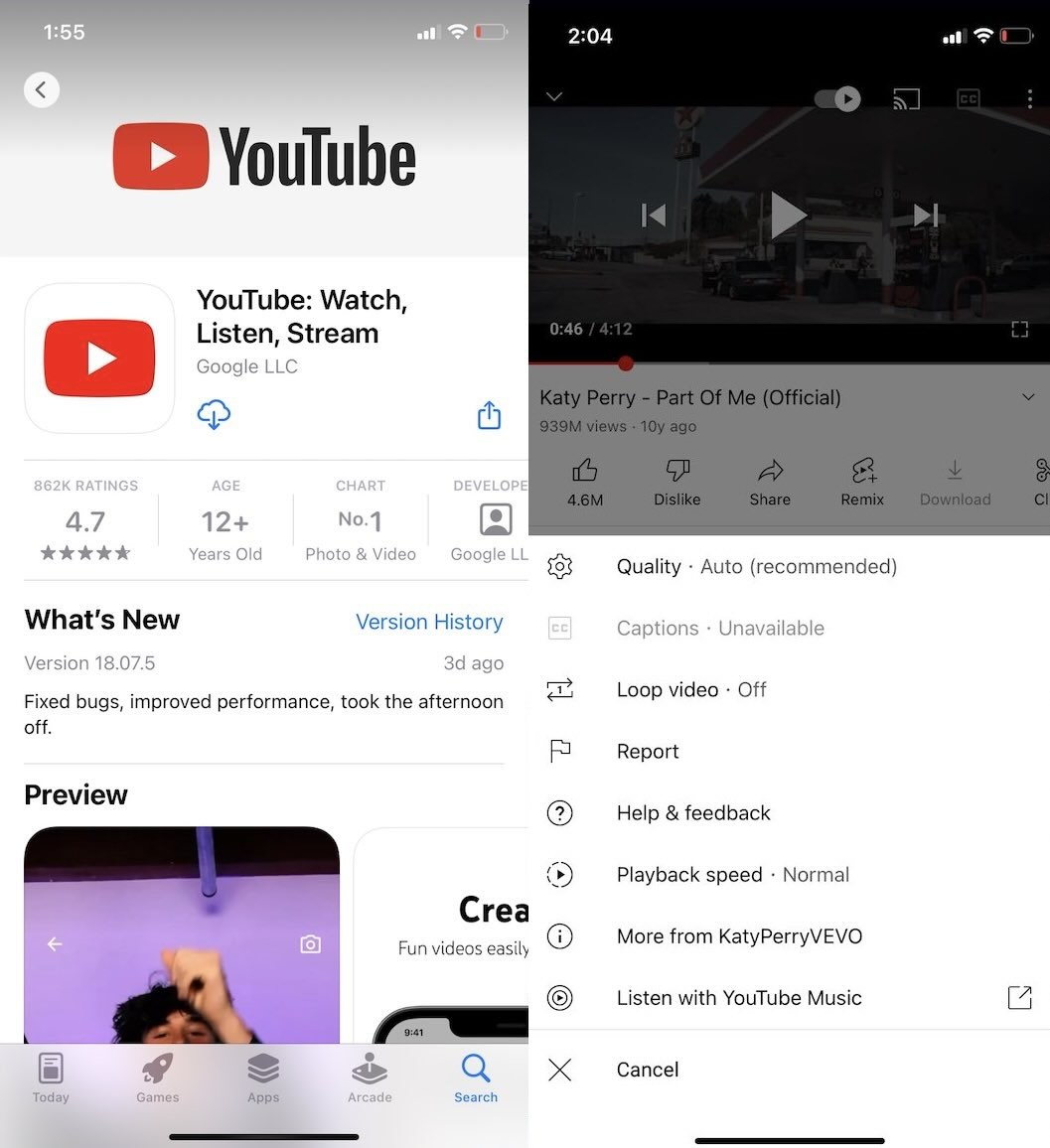The image consists of two separate screenshots, presented side by side in landscape mode, each depicting different stages of interaction with YouTube on a mobile device. 

On the left side of the image:
- The screen displays a YouTube app details page in the App Store.
- The battery indicator shows a low charge, and the time reads 1:55 PM.
- The screen presents two columns of content. At the top, it shows "YouTube" followed by "YouTube: Watch, Listen, Stream."
- A "What's New" section details the latest update which mentions bug fixes, performance improvements, and a playful note about taking the afternoon off.
- Below, there's a preview section featuring a video titled "CREA: Fun Videos Easily."
- The page suggests that the user is scrolling, evidenced by cut-off content at the bottom indicating more to view.

On the right side of the image:
- The screenshot was taken nine minutes later, at 2:04 PM.
- It shows a YouTube video in watch mode, with a prominent play button displayed in the center.
- In the lower-left corner, it indicates that the current video playback is at 46 seconds out of a total of 4 minutes and 12 seconds, with a red dot marking this position on the progress bar.
- The video is the official version of "Part of Me" by Katy Perry, released 10 years ago.
- Additional options under the video include quality settings (set to auto), a loop video option, and links to more content by Katy Perry and "Listen with YouTube Music."

This comprehensive and detailed caption encapsulates both the content and context of the images accurately.